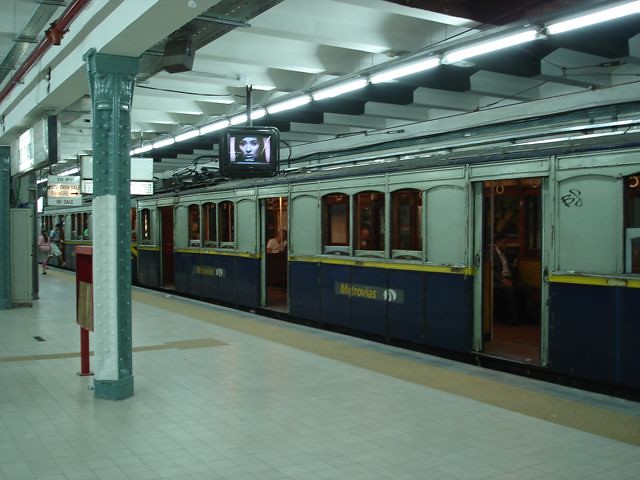This image captures a pristine subway station with a white tiled floor and a white ceiling. A mint green column stands prominently on the left side, complemented by an array of dark and light green pillars throughout the station. Hanging from the ceiling near the column is a black-framed TV displaying the grayscale face of a woman. 

To the right, there's a subway car characterized by a white top, a yellow stripe, and a navy blue bottom. Accompanying this is a tan stripe along the train's side. The subway also features typical windows and doors, with slight graffiti visible near the middle right-hand side. A red newsstand is situated next to one of the green pillars.

The station appears mostly empty, save for a few figures in the far background, including a man seemingly stepping onto the train. The scene is illuminated by the clean, tiled surroundings and shadows cast by overhead signs, reinforcing the station's orderly and well-kept appearance.